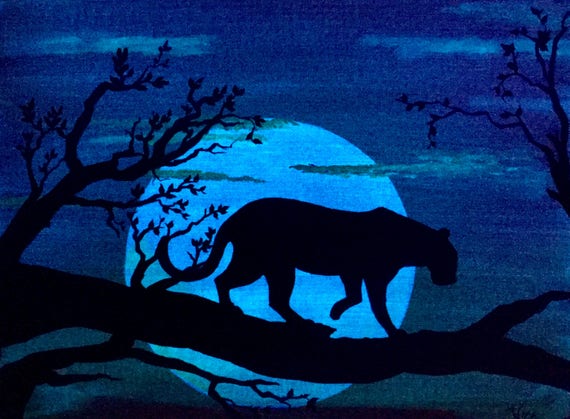This is an aged illustration, possibly from a children's book, portraying a nighttime scene with a black panther, or perhaps a jaguar, walking across a large, thick tree branch extending horizontally from left to right. The panther's silhouette is clearly visible, with its long tail curled up and one left paw lifted as if in mid-step. Above and around the panther, several smaller branches jut upward, adorned with leaves, yet all details remain in solid black without any facial features visible. A vast, pale blue full moon occupies the center of the composition, casting a faint glow that enhances the silhouette of the panther. This moon is set against a dark blue night sky, interspersed with thin, horizontal white clouds. The entire scene evokes a serene yet mysterious nighttime ambiance.